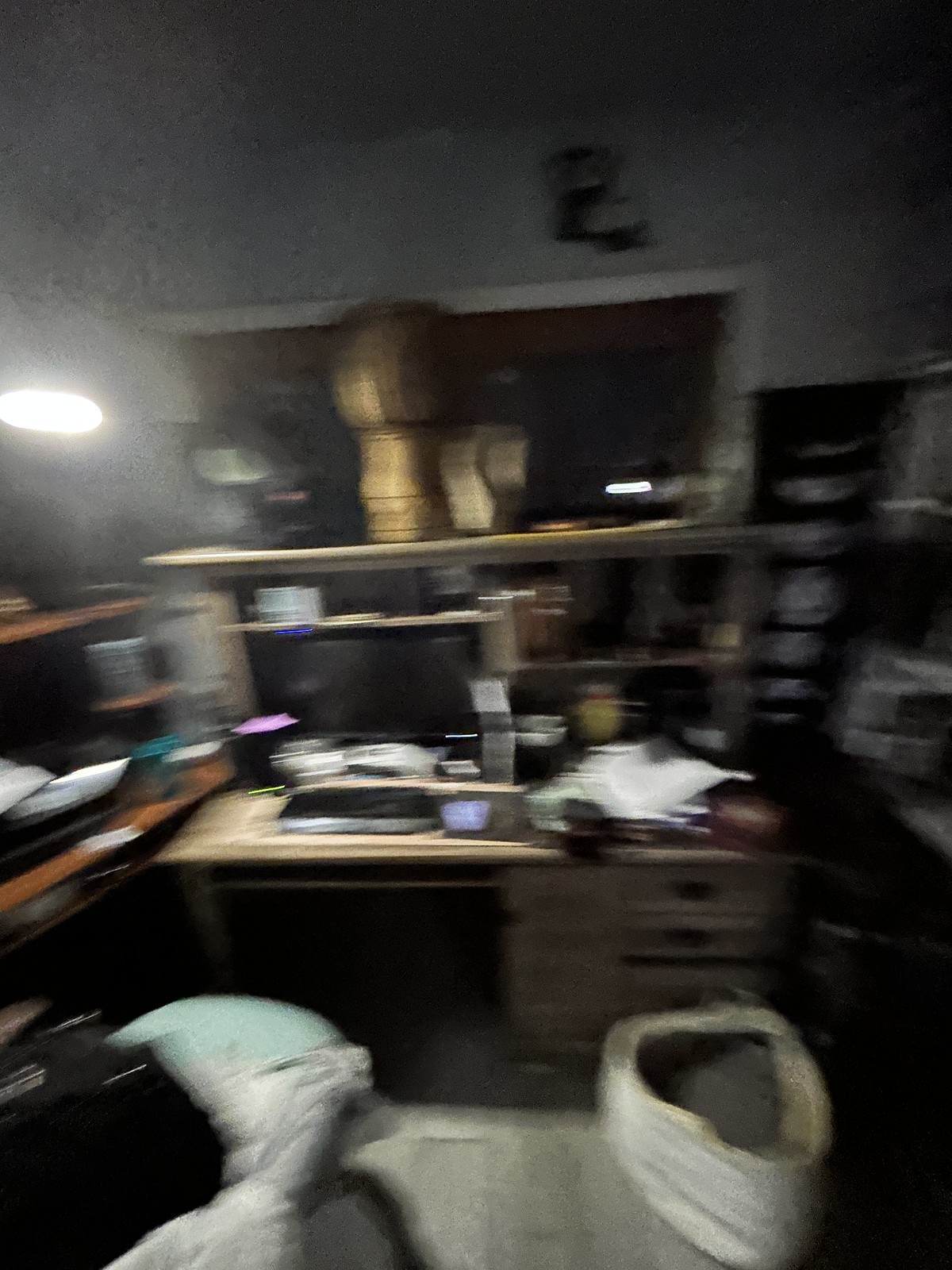This image, although quite blurry, depicts a work desk in a somewhat dimly lit room. The desk appears to be made of wood and features a dual-level structure, with a main surface and an elevated shelf. On the left-hand side, a desk lamp with an exposed bulb provides illumination, though its exact shape is indiscernible. A black computer monitor and keyboard occupy the left side of the desk, while a stack of papers and various trinkets clutter the right side. To the far right, underneath the desk, there are multiple drawers, with a white basket positioned in front of them, possibly serving as a pet's resting spot. The background reveals a large doorway framed with white trim, against what seems to be a light blue wall. In the lower left-hand corner of the image, a chair with a coat draped over its back can be observed.